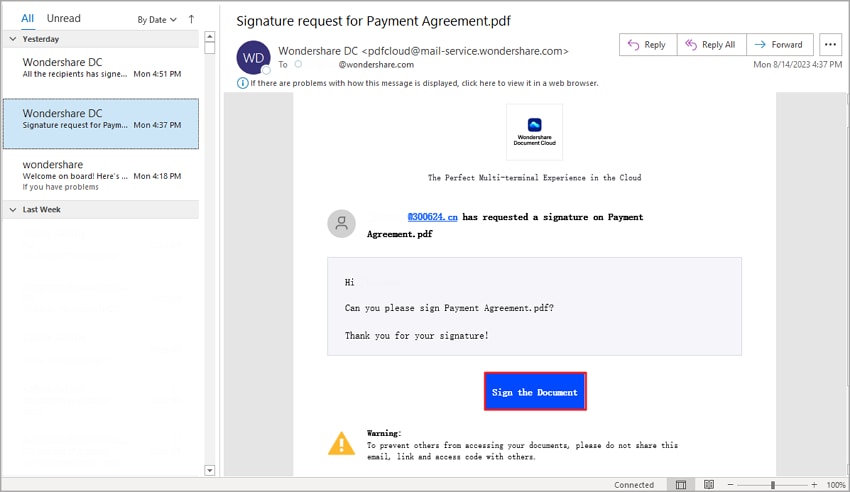This image is an email interface from a website. On the left, a menu shows various email categories. The "All" category is highlighted in blue, indicating it is currently selected. Under the "Yesterday" header, there are two emails from Wondershare DC and one from Wondershare. The primary email displayed is titled "Signature request for payment agreement PDF."

On the right, the interface offers several options for handling the email, including "Reply," "Reply All," "Forward," and an additional options menu represented by three dots. Below these options, the date and time of the email are displayed. The sender's profile picture is a purple icon with the initials "WD" in white letters.

The body of the email features a highlighted section from Wondershare Document Cloud, marked by a blue and dark blue icon. It promotes "The perfect multi-terminal experience in the cloud." At the bottom, there is a prominent blue and red-outlined button labeled "Sign the document." Accompanying this is a warning sign—a yellow triangle with an exclamation point inside—suggesting caution. Additionally, there is a "Connected" button visible in the email body.